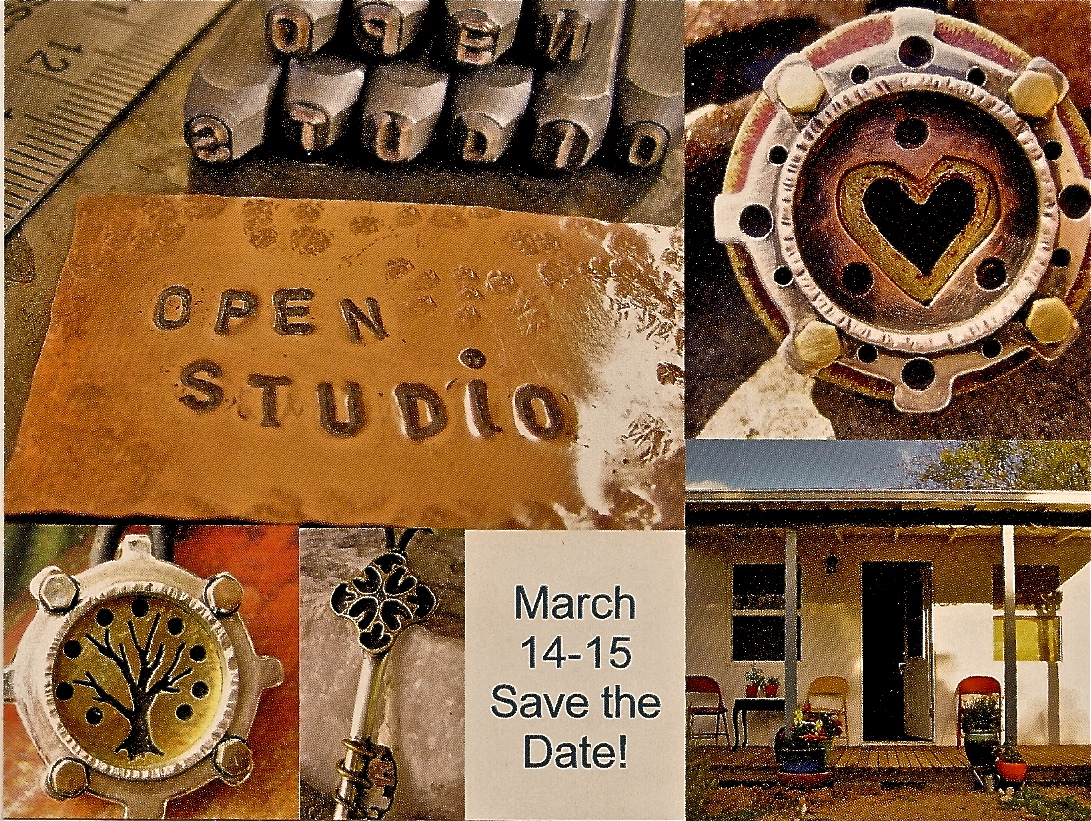This postcard features a collection of four color photographs in a landscape orientation, each showcasing unique elements tied together with a "Save the Date" reminder for March 14-15. The top left photograph, the largest, prominently displays a sign reading "Open Studio," adorned with a ruler and metal bars on top, lending an industrial feel. Below the sign, a brown, glossy clay plate bears the same text, with visible fingerprint indents adding a tactile quality. The top right photograph captures a metallic gear-like object or brake drum with a heart cut-out in its center. The bottom left image displays a similarly shaped metallic circle, this time featuring an artistic imprint of a tree with dots, possibly signifying growth or nature within an industrial context. Beside it is an insignia resembling a key. In the bottom center, a beige box with black text reads "March 14-15, Save the Date!" To the bottom right is a charming, realistic photograph of a white, single-story building with a gabled roof and a welcoming wooden porch. The porch features three chairs, a table, plants, and an open doorway, exuding a cozy and inviting atmosphere. Overall, this postcard blends realism with graphic design, serving as a visually appealing reminder of an upcoming event.